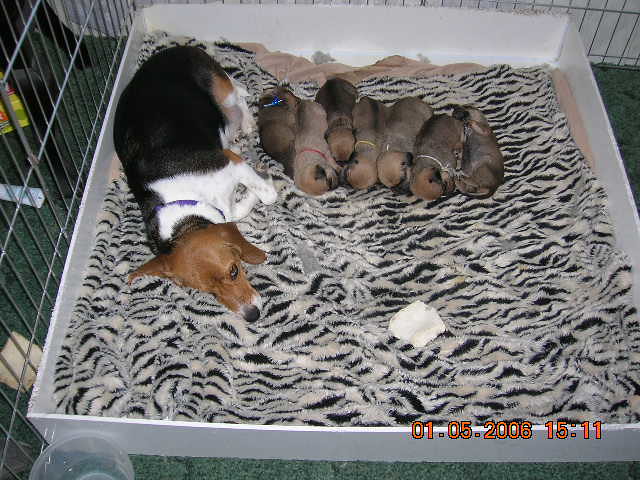In the center of this overhead photograph from January 5, 2006, at 15:11, a large beagle-like dog lies in a white plastic square pen, looking towards the camera. The pen is lined with a zebra-striped black and white blanket. To the right of the mother dog, seven tiny, light brown puppies with tan fur on their heads and black fur around their ears are nestled side by side. The pen is enclosed by a silver metal fence, and it rests on a dark forest green shag carpet. The mother dog has a predominantly black body, a brown head, and white fur along her stomach, with a blue collar around her neck. The date in retro orange font is visible in the bottom right corner of the image.